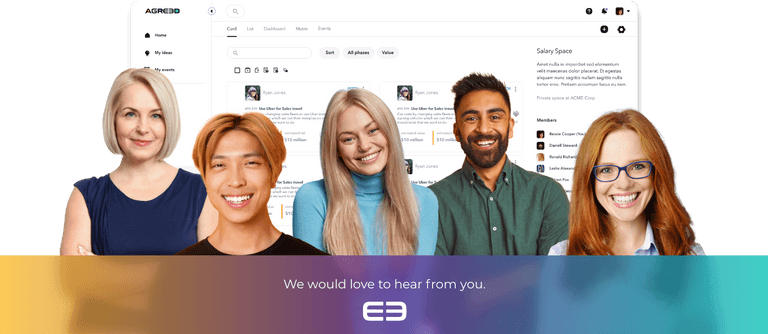The image shows a group of five people posing cheerfully in the foreground against a backdrop of a grid-like website interface. 

From left to right, the individuals include:
1. A female with long brown hair wearing blue glasses and a powder blue shirt.
2. A male in a dark green t-shirt.
3. A female in a blue polo neck shirt.
4. A male in a black t-shirt.
5. A female in a purple dress.

Their heads are at the top of the image while their chests are below, partially covered by a semi-transparent text overlay. The text, written in white, reads "We would like to hear from you." This text is set against a multi-colored background consisting of blue, purple, green, and brown hues, which allows the people behind it to remain visible. 

In the background, the website has a white interface with a grid layout and various images of people scattered throughout. The name "Grid" is displayed in the top-left corner within a black box, while the top-right corner features the text "Salary Space" along with some other unreadable text. 

The overall scene captures a blend of cheerful human interaction and digital interface, emphasizing engagement and communication.